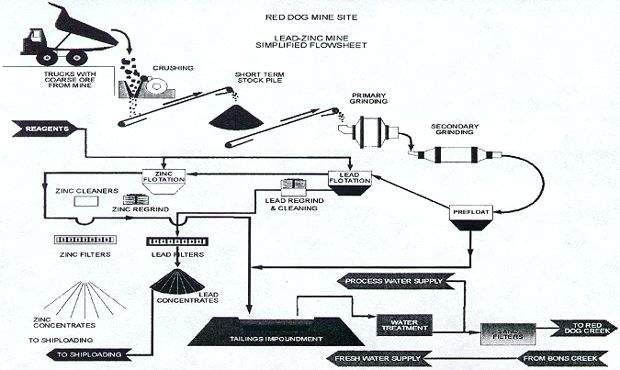This image showcases a detailed flow chart diagram titled "Red Dog Mine Site: Lead Zinc Mine Simplified Flow Sheet," set against a white background. At the top left, a truck is depicted dumping coarse ore from the mine, which undergoes sequential processes starting with crushing. The ore is then stored in a short-term stockpile before moving through primary and secondary grinding phases. Following grinding, the flow sheet delineates several stages of separation and purification: lead flotation, lead regrind and cleaning, zinc flotation, zinc cleaners, zinc regrind, and both lead and zinc filters. Finally, the diagram shows the extraction of lead and zinc concentrates, which are subsequently prepared for ship loading. Fresh water supply is also integrated into the process, highlighting its role in the mining operation. The entire flow sheet visualizes the cyclical and methodical approach of processing lead and zinc ores at the Red Dog Mine Site.